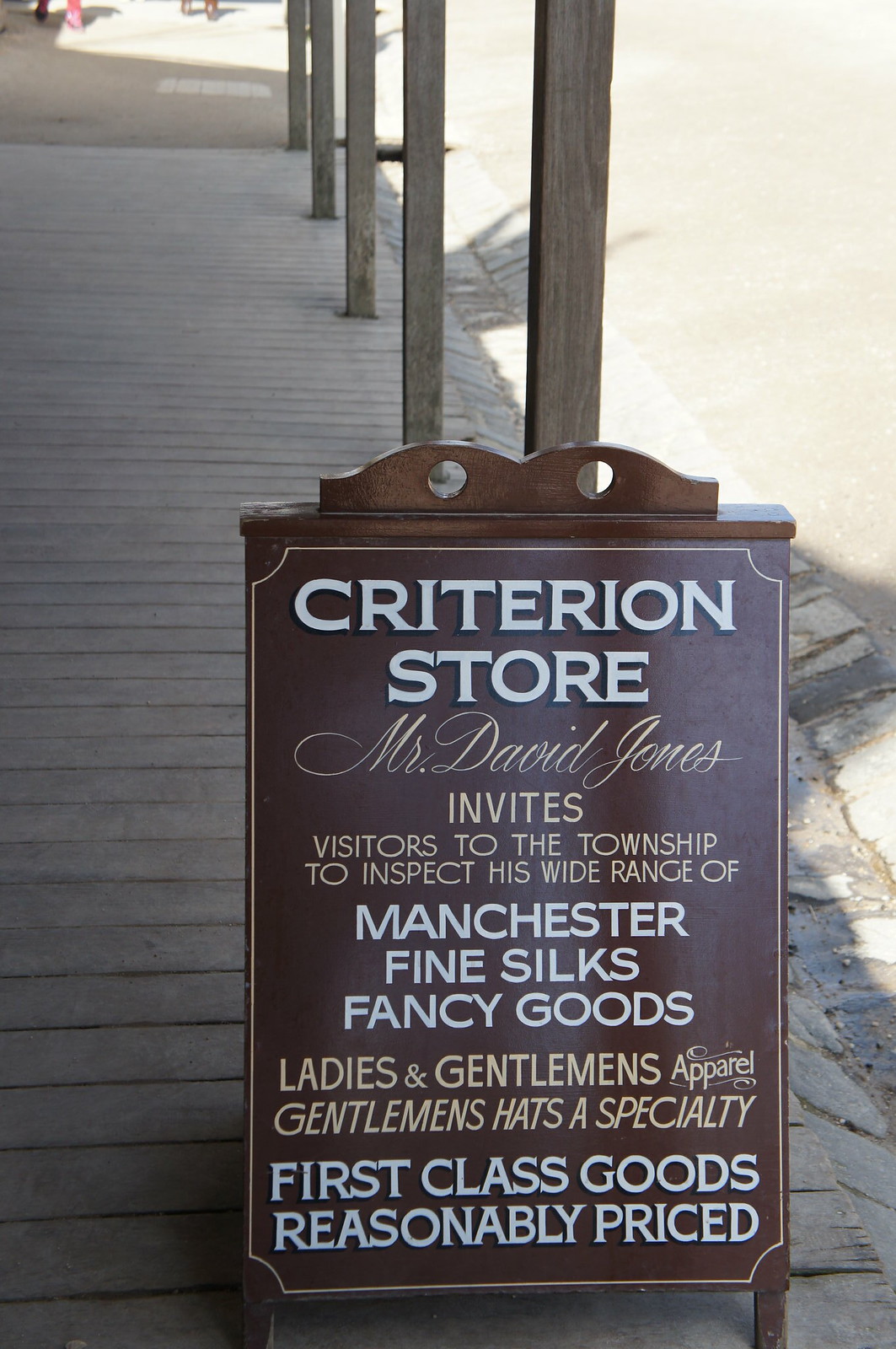In the image, we see an Old West-themed scene characterized by vintage wooden buildings, complete with wooden floors and pillars. At the front, just before reaching a sandy dirt road, there's a detailed wooden sign leaning against one of the posts on a wooden deck. The sign, primarily brown, features a combination of fonts and colors. It prominently displays "Criterion Store" in large, white lettering at the top. Below, in a cursive, tannish-gold font, the proprietor, Mr. David Jones, invites visitors to explore his varied selection. The offerings include "Manchester Fine Silks Fancy Goods" in white letters, "Ladies and Gentlemen's Apparel" and "Gentlemen's Hats a Specialty" in a lighter brown color, and finally, in bold, uppercase white font, "First Class Goods Reasonably Priced." This meticulously crafted sign tells us that the store specializes in high-quality Western clothing and accessories, and adds a historical charm to the outdoor setting captured during the daytime.